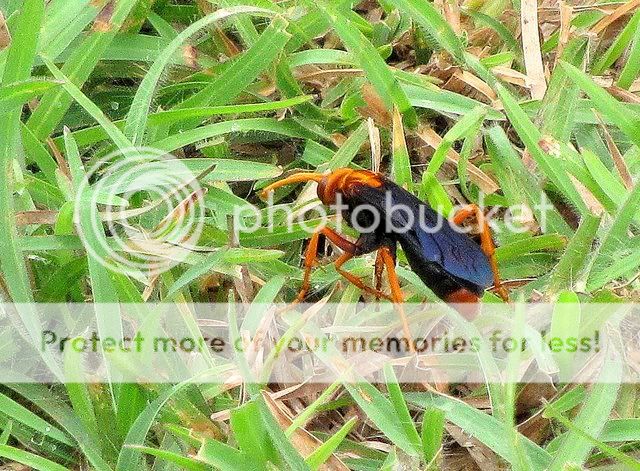This image, sourced from Photobucket, features an extreme close-up of a large black and yellow wasp positioned on top of blades of grass. The insect’s body is a striking yellow-orange, transitioning to black wings, with its head and legs also showcasing a golden orange hue. The wasp is depicted walking across a patch of grass, where both dead and living blades are visible, indicating a garden or field environment. The texture of the grass is detailed enough to reveal individual hairs. The wasp is oriented towards the top-left corner of the frame. The entire image is partially obscured by multiple watermarks, including a semi-transparent circular overlay with the Photobucket logo and a white box containing the text “Protect more of your memories for less.”